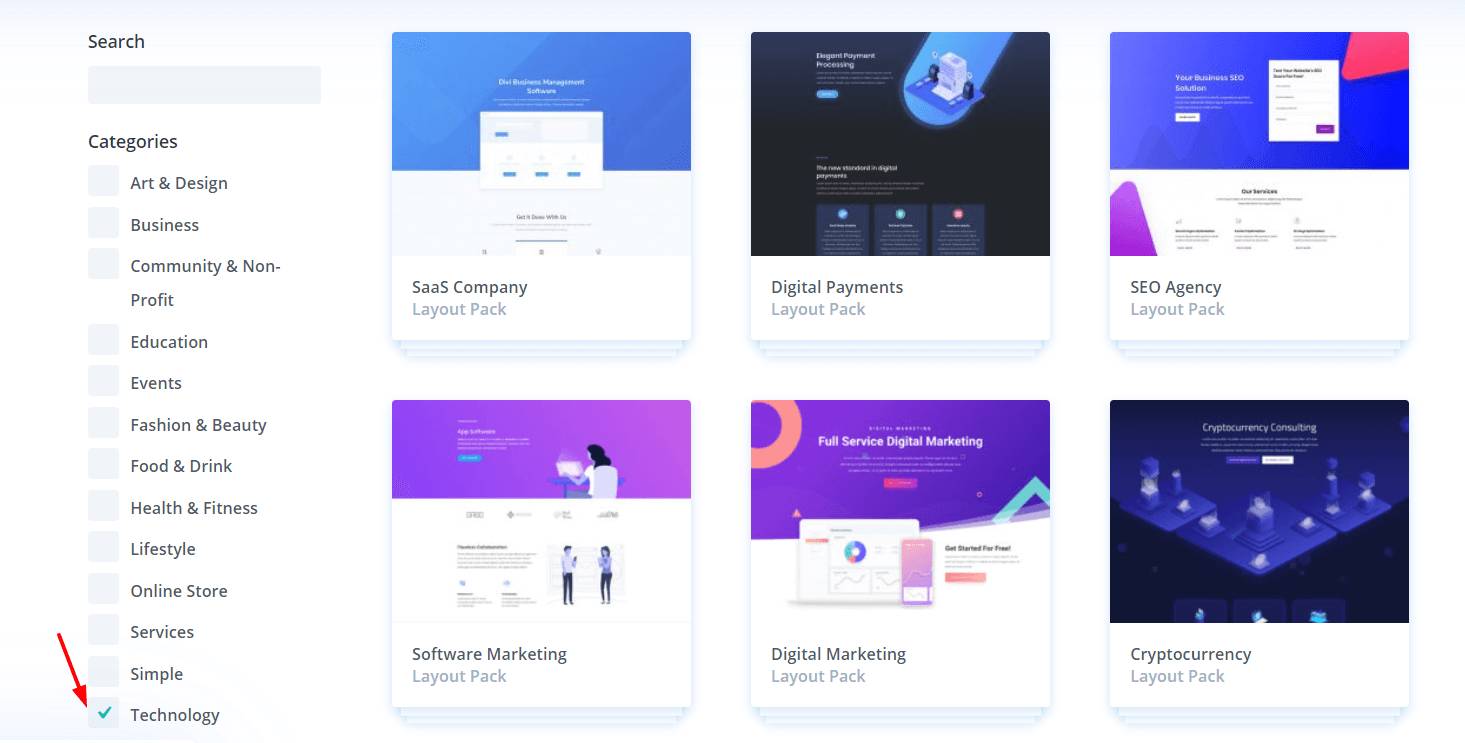The image depicts a section of a website dedicated to creating websites. On the left-hand side, there is a search bar positioned at the top-left corner. Below the search bar, a list of categories is displayed in a vertical fashion. The categories are: Art and Design, Business, Community and Non-profit, Education, Events, Fashion and Beauty, Food and Drink, Health and Fitness, Lifestyle, Online Store, Services, Simple, and Technology. The 'Technology' category is selected, with a red arrow pointing towards its checkbox.

On the right-hand side, there are six tiles arranged in two rows, each showcasing a different layout pack available for selection. Each tile has the words "Layout Pack" written in grey text beneath its headline. The first tile in the upper row is labeled "SAAS Company," featuring a blue and white background. The second tile, "Digital Payments," has a predominantly black background with blue accents. The third tile, "SEO Agency," is divided halfway with blue and white colors, accompanied by some text.

In the lower row, the first tile is labeled "Software Marketing" with a purple and white theme. The second tile, "Digital Marketing," is also purple and white and includes some graphical elements. The last tile, titled "Cryptocurrency," features a dark black or blue background with blue accents. Each tile represents a distinct website layout pack available for users to choose from within the 'Technology' category.